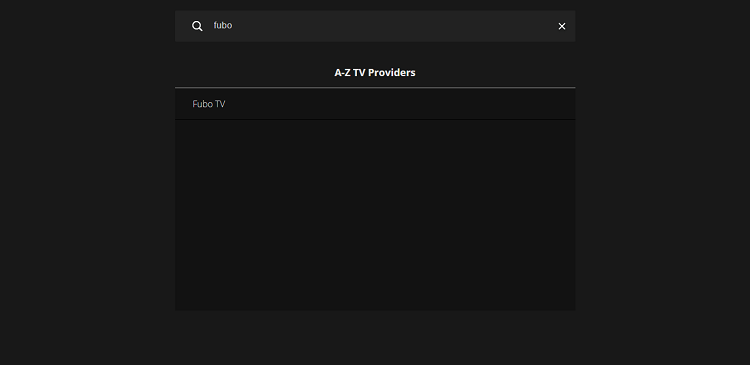In the image, a person is browsing TV providers. The search bar at the top displays the term "Fubo" against a light gray background. Below the search bar, the title "A to Z TV Providers" is prominently displayed in white font. The name "Fubo TV" is listed beneath this title, also in white letters, contributing to the contrast. The central portion of the image is dominated by a large black rectangle, slightly offset against a marginally lighter dark gray background. This composition accentuates the focus on the content displayed. The surrounding elements are minimal, ensuring that attention remains fixed on the search results for Fubo TV. The use of varying shades of black and gray creates depth and guides the viewer's eye to the essential information in the center.